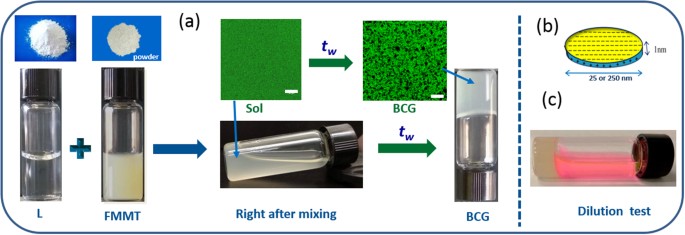This image appears to be a detailed diagram, possibly from a biology or chemistry educational presentation, illustrating a sequence of chemical mixing and testing processes. On the left, there is a rectangular area with rounded corners outlined in blue, containing multiple sections. At the top left is a blue rectangle with white powder on it, next to another blue rectangle with a smaller amount of white powder. Below these rectangles are two small bottles, labeled 'L' and 'FMMT,' with a plus sign between them. 

The first bottle is entirely grey, while the second has a grey top and a cream-colored bottom with an arrow pointing downward, marked with '(A)'. To the right, there's a green square containing a small white rectangle and labeled 'SOL,' next to a green arrow pointing rightwards beneath purple text reading 'T' and 'W.' Adjacent is another green square, appearing to depict plants, labeled 'BCG.' 

Underneath the first green square, an image of a tilted jar with a blue arrow coming from the green square and labeled 'right after mixing' is displayed. Another arrow marked 'TW' and showing a green solution connects to a second jar, now upright, still interacting with the green square labeled 'BCG.' A vertical slash line separates sections, leading to a yellow-filled blue container with a downward arrow stating '25 or 250 nm,' followed by a double arrow indicating '1mn,' and labeled '(B).'

The diagram concludes with a depiction of another bottle lying sideways, this one containing a pink substance, labeled 'dilution test'. This comprehensive diagram appears to demonstrate the steps of adding chemical powders into vials, observing the resulting mixtures immediately after combining, and performing a dilution test to examine the changes.